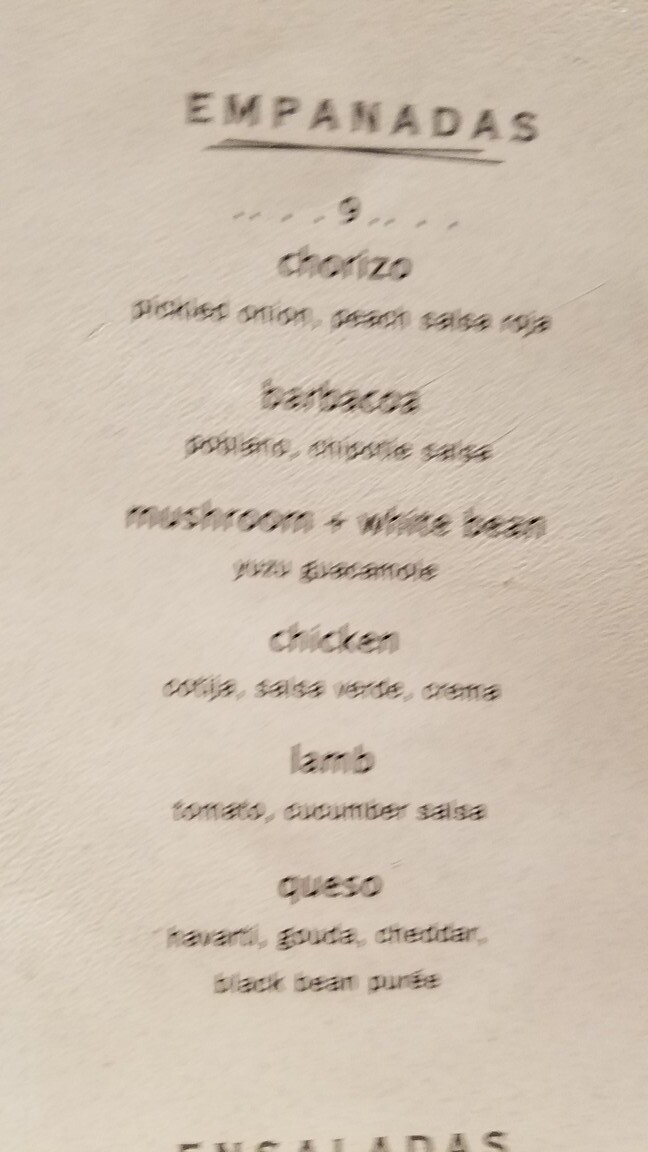An image captures a detailed menu of empanadas, presented against a beige background. The title "Empanadas" is displayed prominently in bold black text, indicating each is priced at nine dollars. The menu lists a variety of empanada flavors: chorizo, barracuda, mushroom and white bean, chicken, lamb, and queso. Underneath each flavor, there are additional details, such as the lamb empanada, which is accompanied by a tomato and cucumber salsa. The photo, although slightly out of focus, allows for the primary information to be discernible. At the bottom of the image, there is a glimpse of another menu item, possibly enchiladas, but it is partially cut off. Two black lines form a crisscross pattern beneath the empanada listings. The focus issue slightly obscures finer details, but the main elements of the menu are still recognizable.